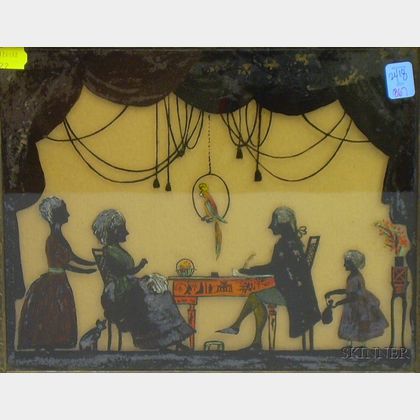The photograph captures an 18th-century styled stage scene, reminiscent of a shadow box, likely on display at a garage sale. Encased behind glass, the scene is surrounded by black fabric curtains giving it a theatrical aura. Central to the display is a brown wooden table, where a man resembling George Washington or Thomas Jefferson sits with a quill, appearing to write, opposite a woman with a voluminous hairdo. Both are adorned in colonial attire; the man wears a white wig with a ponytail, a frock coat, knee-high shorts, and leggings, while the woman is in an ankle-length puffed dress. Around them, a young girl and a servant, both in mop caps and old-fashioned dresses, contribute to the historical atmosphere. Above the table hangs a parrot on a ring. The characters, although in silhouette against a yellowish backdrop, display subtle clothing colors—hints of blue, gray, and red, adding depth to this intricate depiction of an 18th-century tableau.